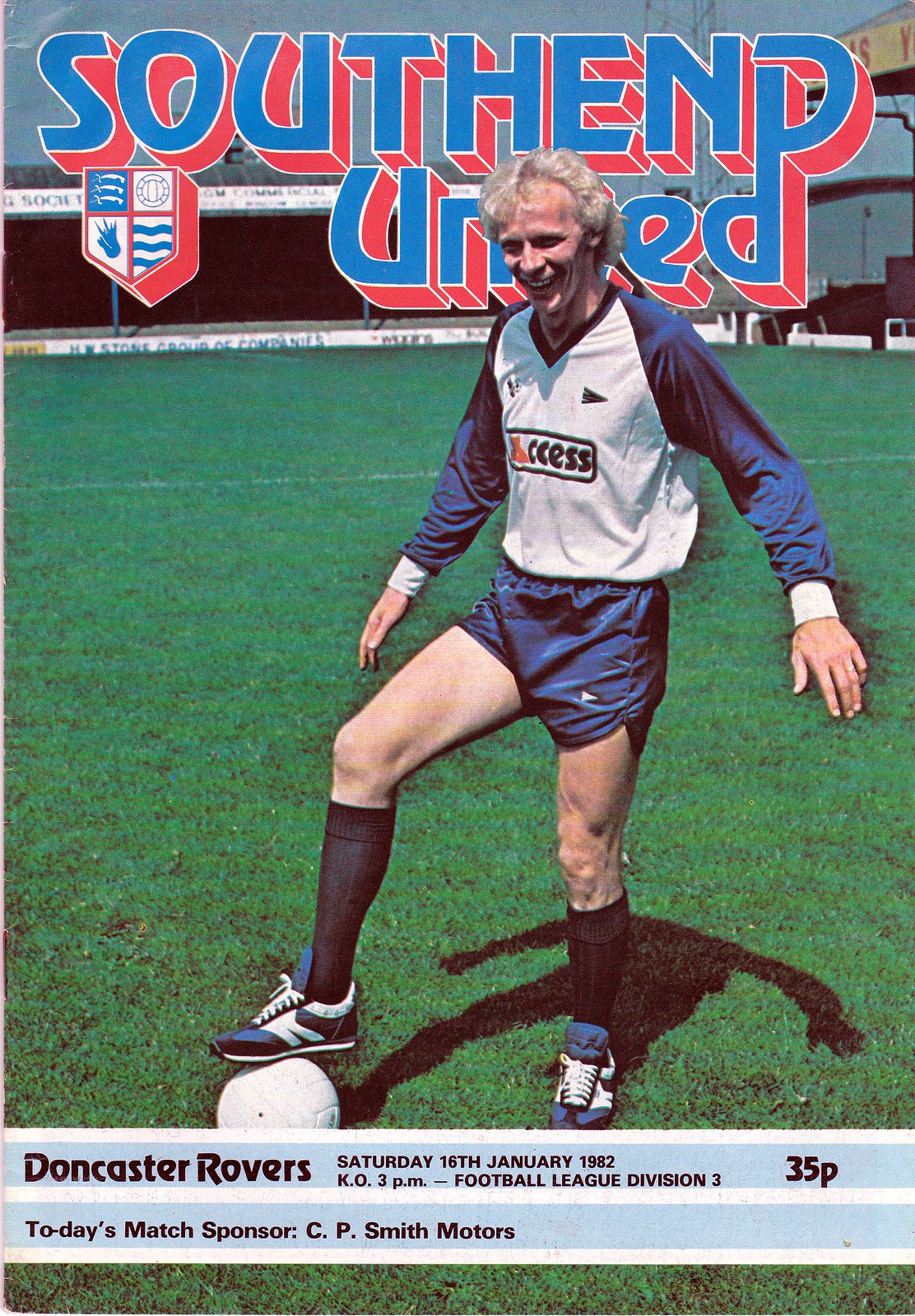This image is the cover of a soccer program for a match between South End United and Doncaster Rovers, scheduled for Saturday, January 16th, 1982, with a 3 p.m. kickoff in the Football League Division 3. The program is sponsored by C.P. Smith Motors, and the cover price is listed as 35p. At the top of the cover, the title "South End United" is prominently displayed in blue and red letters, alongside the South End United logo, which features a distinctive square with a pointed bottom. 

Centrally positioned is a soccer player with pale skin and blonde hair, wearing a blue, white, and red jersey that has the word "Access" on the front, blue shorts, black socks, and blue shoes. The player is standing on the field with his hands outstretched and his right foot resting atop a white soccer ball. The green grass of the well-maintained pitch forms the background for the lower three-quarters of the image, while the top quarter includes additional elements like the South End United logo and informative text. The player is smiling, and his shadow is cast behind him, emphasizing the bright, clear day depicted in this detailed and vibrant soccer program cover.